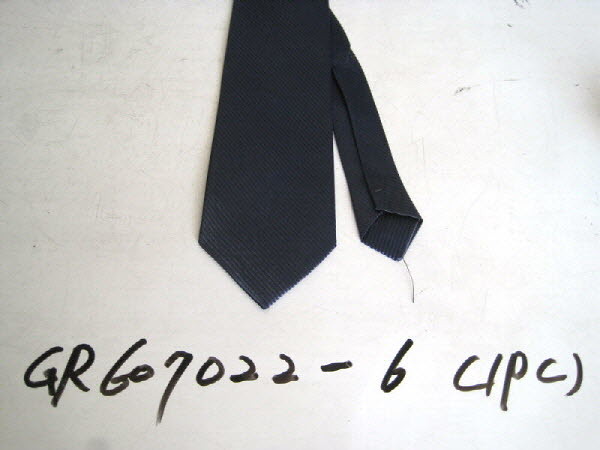The image depicts a solid black tie centered against an off-white background that is noticeably dirty with smudges, thin light grey lines, and black scuff marks, particularly on the top right side. The tie's larger triangular end points slightly to the left, while the smaller triangular end, which reveals its underside, angles slightly to the right. A black thread hangs from the right-hand side of this smaller triangle. Positioned just below the tie is text written in black marker, reading "GR607022-6, (CIPC)." The background also features thin, tannish-grey lines, adding to its textured appearance.